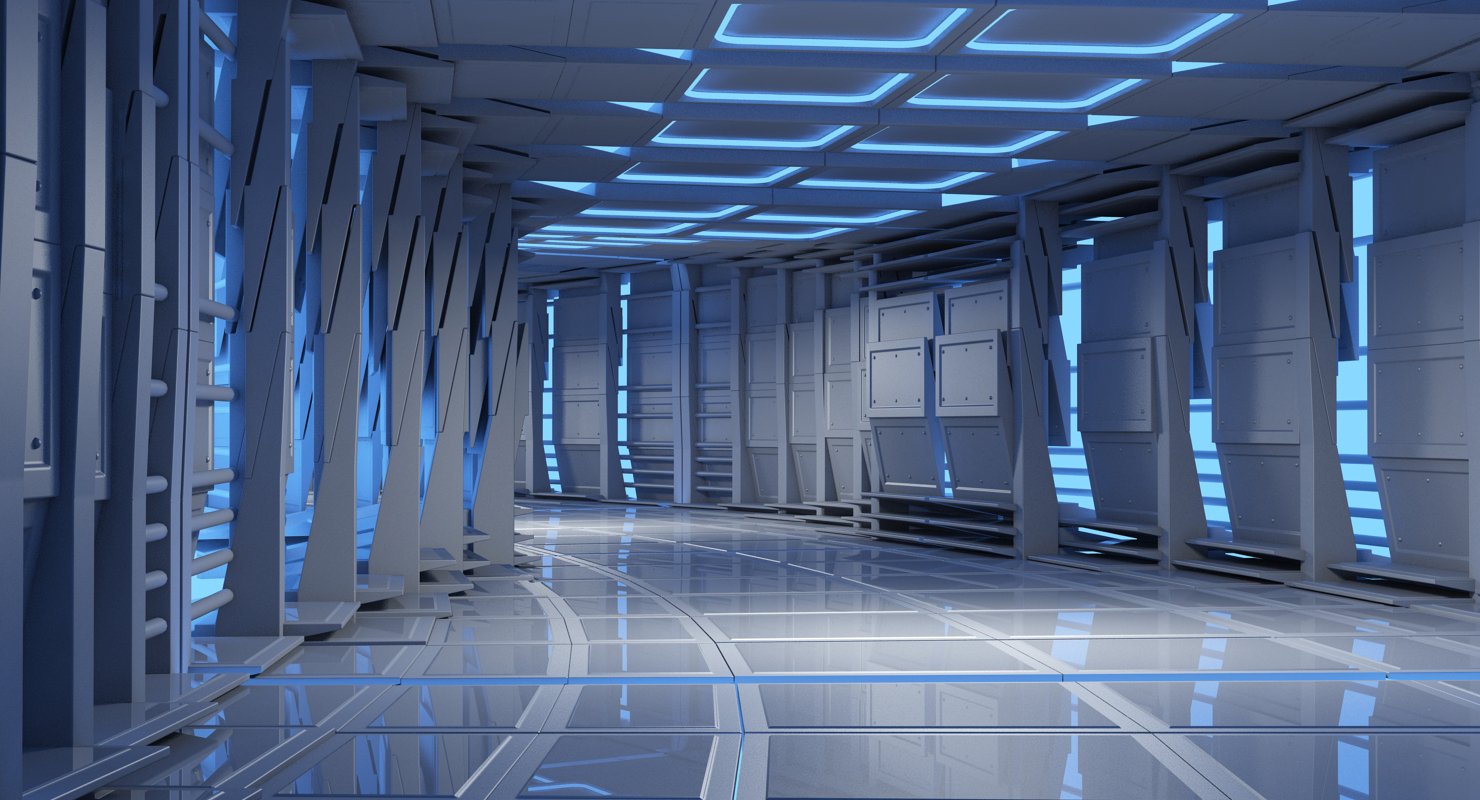The photograph captures a highly polished, futuristic hallway that evokes the atmosphere of a science fiction movie set, reminiscent of the Starship Enterprise or a Star Wars spaceship. The floor is a gleaming silver or shiny white, reflecting the intricate design of the walls and the embedded blue and gray LED lighting. The walls are decorated with multiple rectangular panels, each section featuring a light blue translucent backing with horizontal blue stripes that resemble plexiglass. These panels are arranged in four rectangular sections and are repeated along the wall. Above, the ceiling panels are similarly fitted with embedded blue lights, contributing to the high-tech ambiance. The hallway curves gracefully, reinforcing the sense of being aboard a sophisticated spacecraft. On the left side of the corridor, gray columns—potentially made of metal or plastic—add structure to the scene. The photograph is in color but predominantly features tones of gray and blue, enhancing the futuristic and sterile aesthetic. The space is devoid of any people, robots, or other objects, allowing the viewer to fully appreciate the sleek and expansive design of this science-fiction corridor.